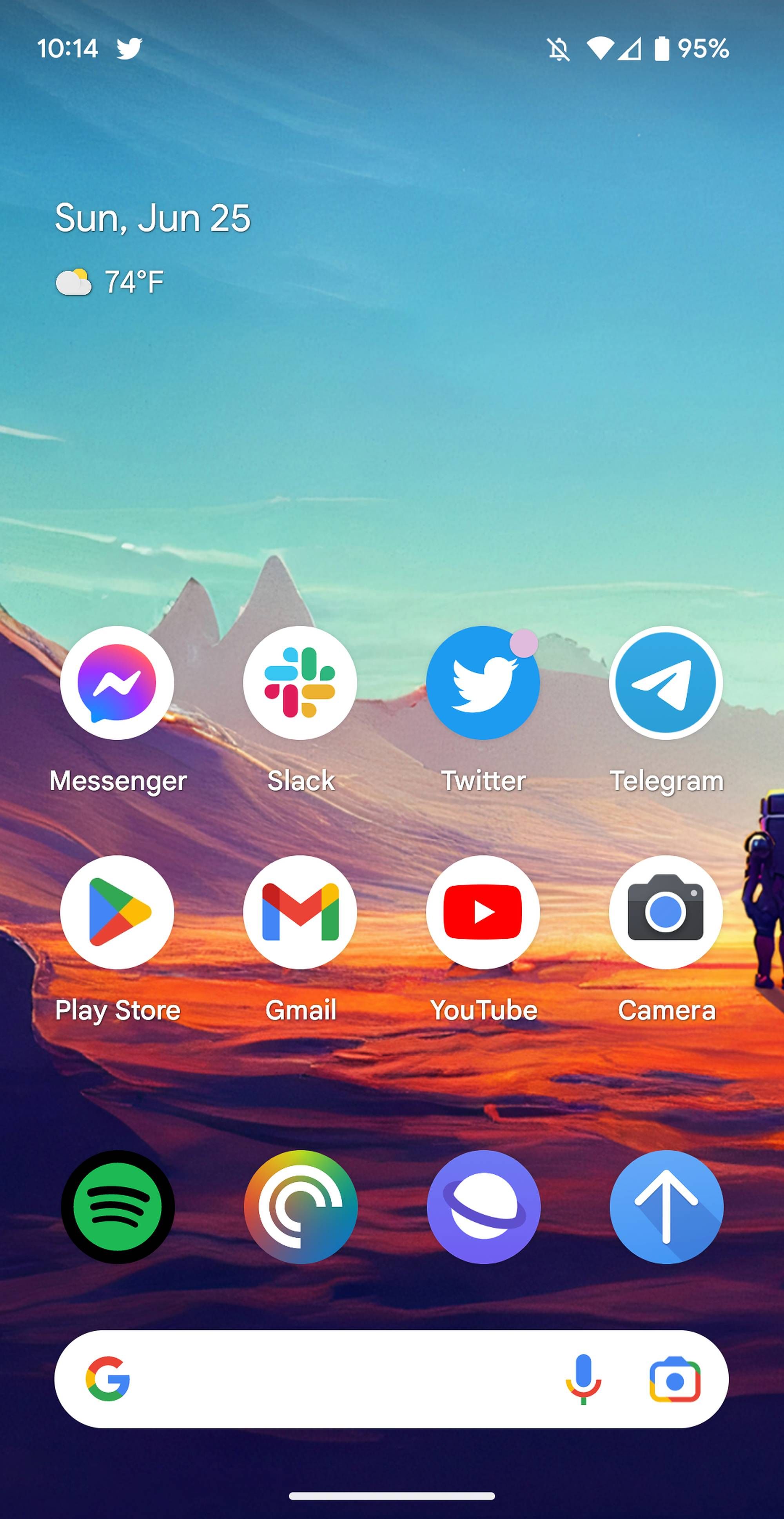A detailed and polished caption for the image could be:

---

The image shows a smartphone screen with a picturesque background and several app icons overlaying it. At the top left corner of the screen, the time is displayed as 10:14. Adjacent to it is the Twitter bird icon, suggesting a notification. Traveling rightwards, a bell icon with a slash through it indicates muted notifications, followed by a Wi-Fi signal icon. Further along, an inverted triangle represents mobile data status, and to the far right, the battery icon reads 95%.

The background image is a bright and sunny day, featuring a clear blue sky with faint hints of yellow, possibly due to a sunrise or sunset. Towering mountains, characteristic of a desert landscape, dominate the horizon. To the far right, near the edge of the screen, a figure in an unusual suit or costume can be seen walking.

The screen displays multiple app icons: Messenger, Slack, Twitter, Telegram, Play Store, Gmail, YouTube, Camera, and another row of unidentified icons below. This setup indicates a well-organized and frequently used smartphone interface.